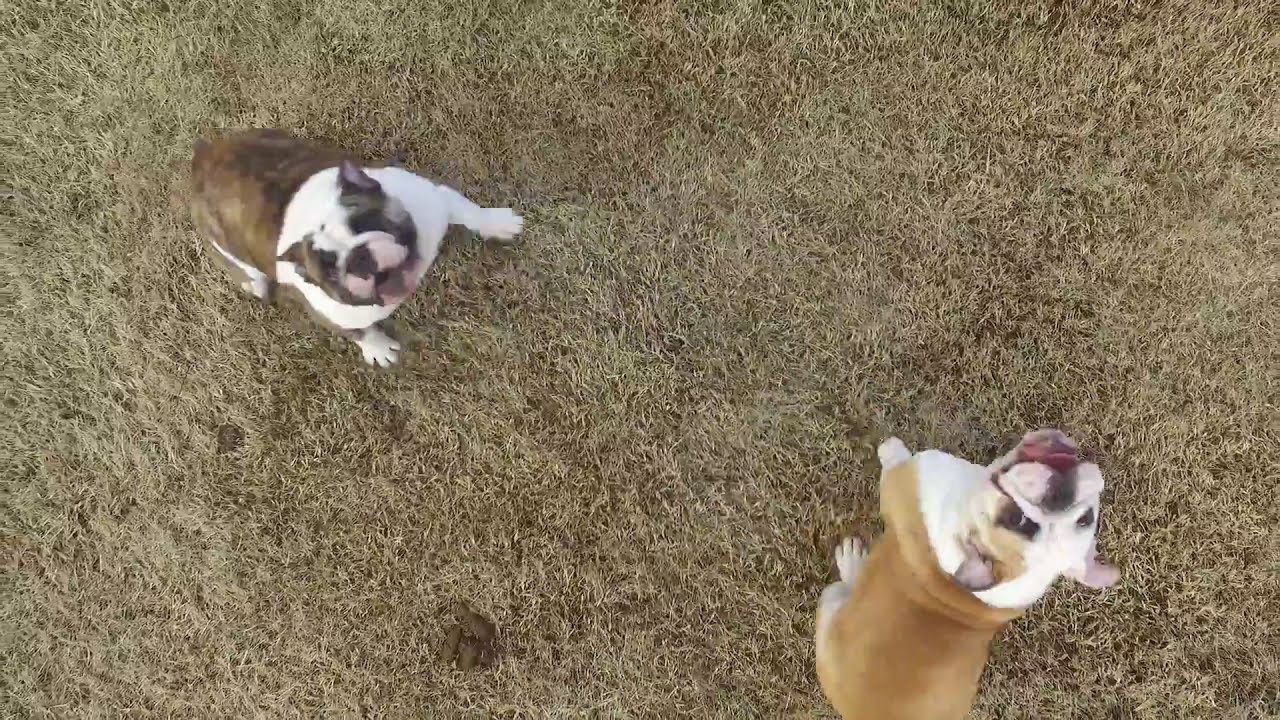The image features two bulldog-like dogs standing on a patch of yellowish, dormant grass, which appears freshly cut and includes a darker brown area with a small pile of poop in the lower center. Both dogs are gazing upwards towards the camera. The bulldog in the upper left corner has a predominantly white body with a darker brown back, pointy ears, and a face marked by a white forehead and snout, with dark patches around the ears and cheeks. The bulldog in the lower right corner displays a light brown body, a white chest and paws, and a white face with a hint of light brown near the left eye.